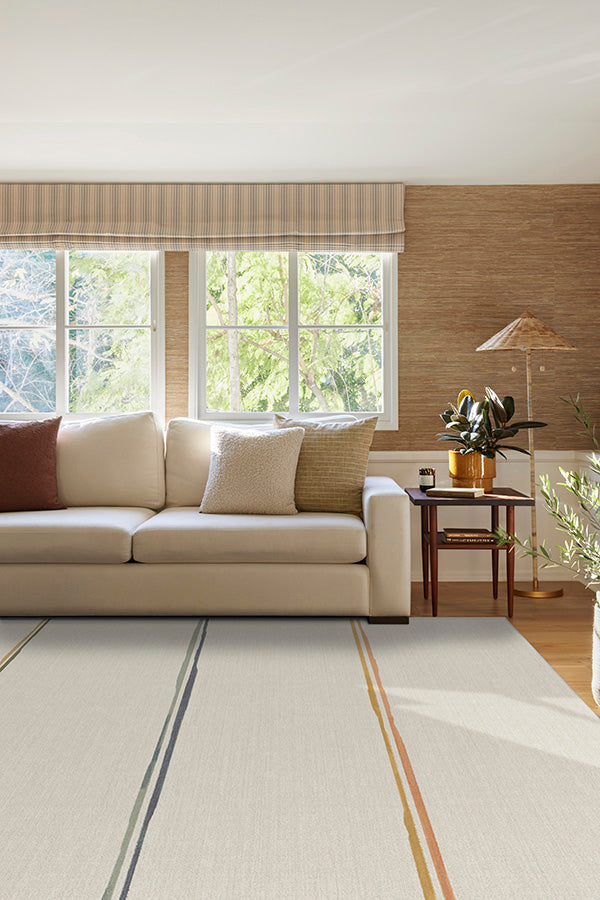The image depicts a professionally styled living room with a modern, elegant design and earthy tones. The room features a large white rug adorned with symmetrical sections and stripes: two and a half feet of plain white, followed by two close golden yellow stripes, then another two and a half feet of white, two bluish stripes, another two and a half feet of white, and finishing with another golden stripe section. A sophisticated white loveseat couch sits against the wall beneath two windows that reveal a verdant, sunlit yard. The couch is complemented with plush cushions, including a fuzzy white pillow and a golden one. The wall behind the couch is two-toned: the bottom half is white and the top half is brown wooden paneling. Beige curtains hang above the windows. An end table next to the couch holds a potted plant in a light brown pot and several books, with another small potted plant nearby. A lamp with an oriental-inspired shade and an earthy, wooden design stands beside the table. The combination of white, beige, and brown elements creates a harmonious and inviting atmosphere.